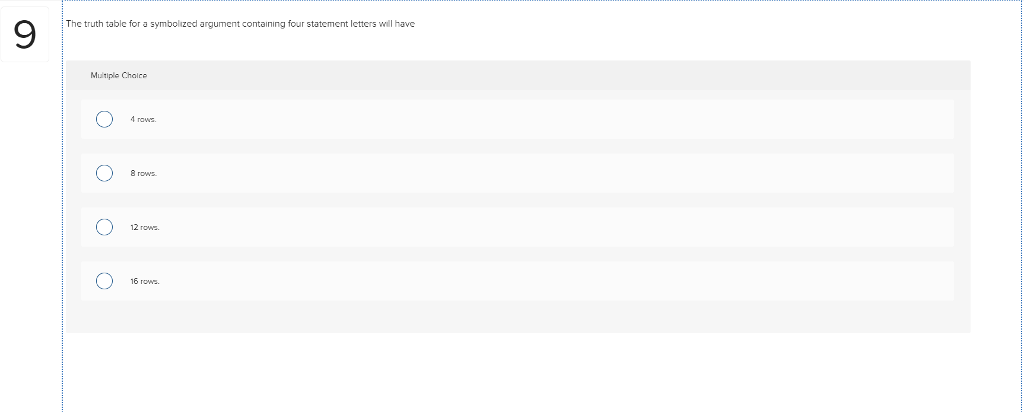The image depicts a computer screen displaying a question from a multiple-choice test. In the upper left corner of the screen, there is a black number "9." Below this, a thin blue outline forms a box containing a question. The question, in black text against a white background, reads: "The truth table for a symbolized argument containing four statement letters will have." The phrase "multiple choice" appears beneath this statement, indicating the format of the question.

Four answer options are listed below the question:

1. Four rows
2. Eight rows
3. Twelve rows
4. Sixteen rows

Each option is preceded by a circle outlined in pale blue, presumably for the user to select their answer. The majority of the screen features a white background, though certain sections, such as the "multiple choice" label and spaces between the answer rows, have a grayish tint. This visual differentiation might serve to distinguish these critical areas from the rest of the content more effectively.